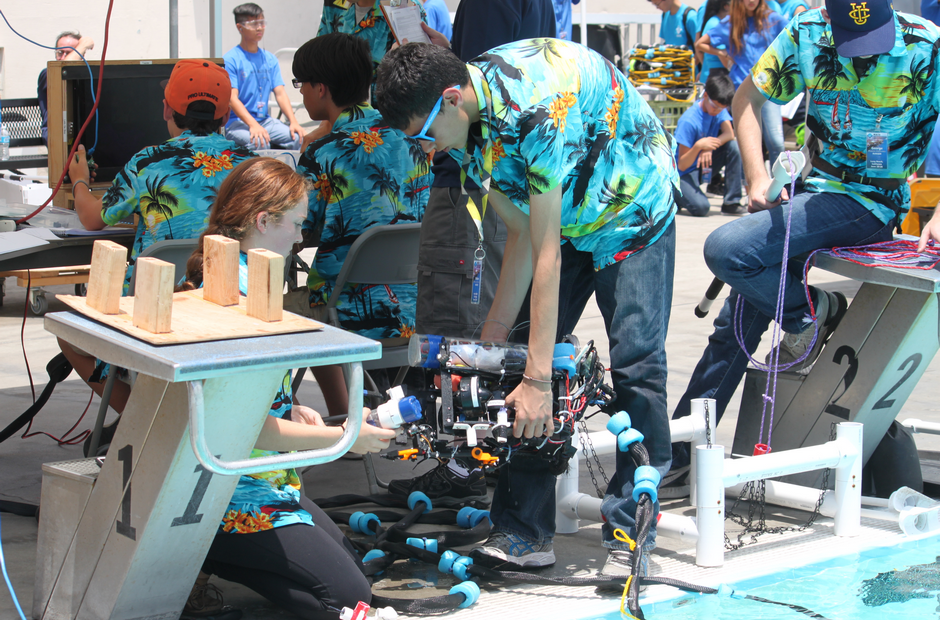This captivating image captures a team of high school students immersed in preparing for the International Robotics Competition at Long Beach City College. At the center of the photograph, a young man, slouching forward towards the left, is intently engaged with a robot, while a young woman, laying on the ground, appears to be fixing an intricate part of the device. Surrounding them are several team members, all donned in matching blue shirts adorned with vibrant Hawaii patterns, including palm trees and orange flowers. Some members also wear lanyards with name tags, indicating their organized involvement in the event. The setting is the diving platforms of a pool, specifically designated with numbered tables—number one on the left and number two on the right, where another man is seen sitting. Scattered around the area are blue foam pieces connected to wires, suggesting the complexity of their project. The youthful energy and collaborative spirit of these young adults highlight their dedication to robotics and their excitement in competing on an international stage.